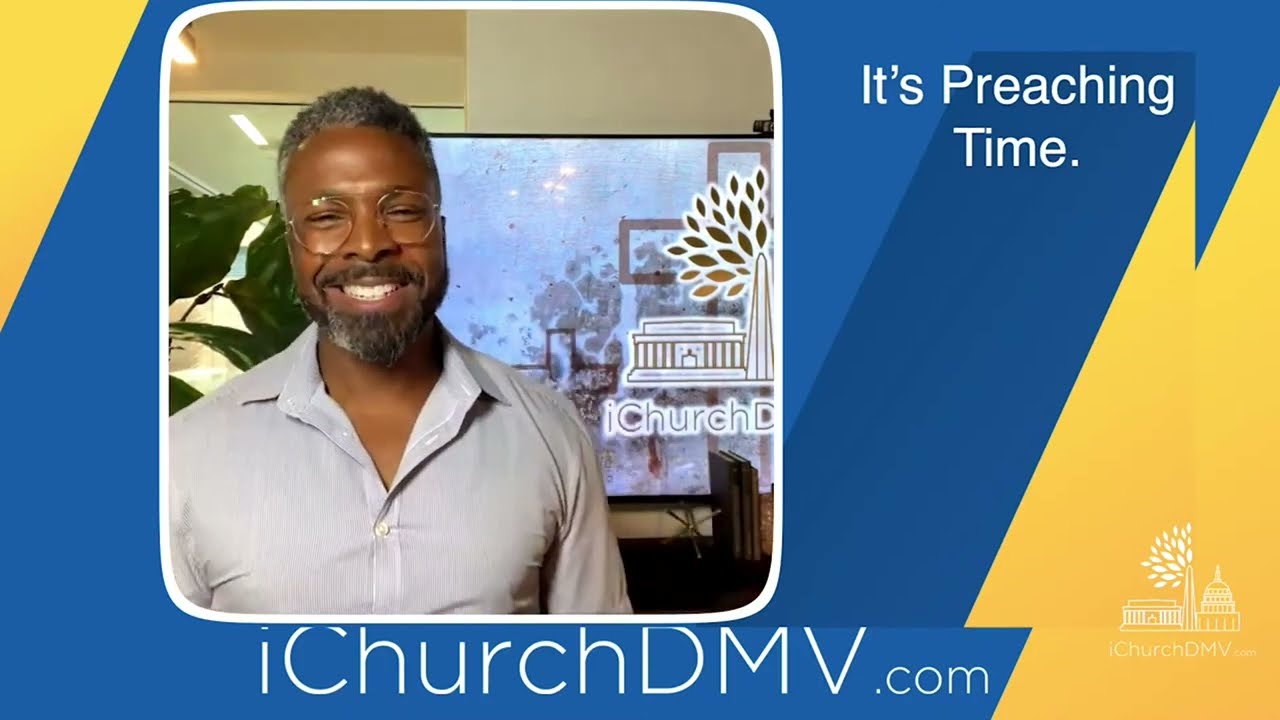This image is an advertisement for a church, featuring a webpage or screen grab showcasing an African-American man, likely in his 50s, who is smiling. He has salt-and-pepper hair, a beard, and mustache, and is wearing clear glasses along with a blue-gray button-up shirt. The background features a mix of light blue, dark blue, and yellow colors.

In the bottom right corner of the image, the church's logo along with the text "iChurchDMV.com" is prominently displayed in white. The same website URL "iChurchDMV.com" is also written in large white letters at the very bottom of the image. Behind the man, there is a TV screen also displaying the church logo, and over his right shoulder, there is a green plant. The upper right corner of the image features the text "It's Preaching Time" in white. The overall setting appears to be indoors, designed to resemble a modern and welcoming advertisement for the church.